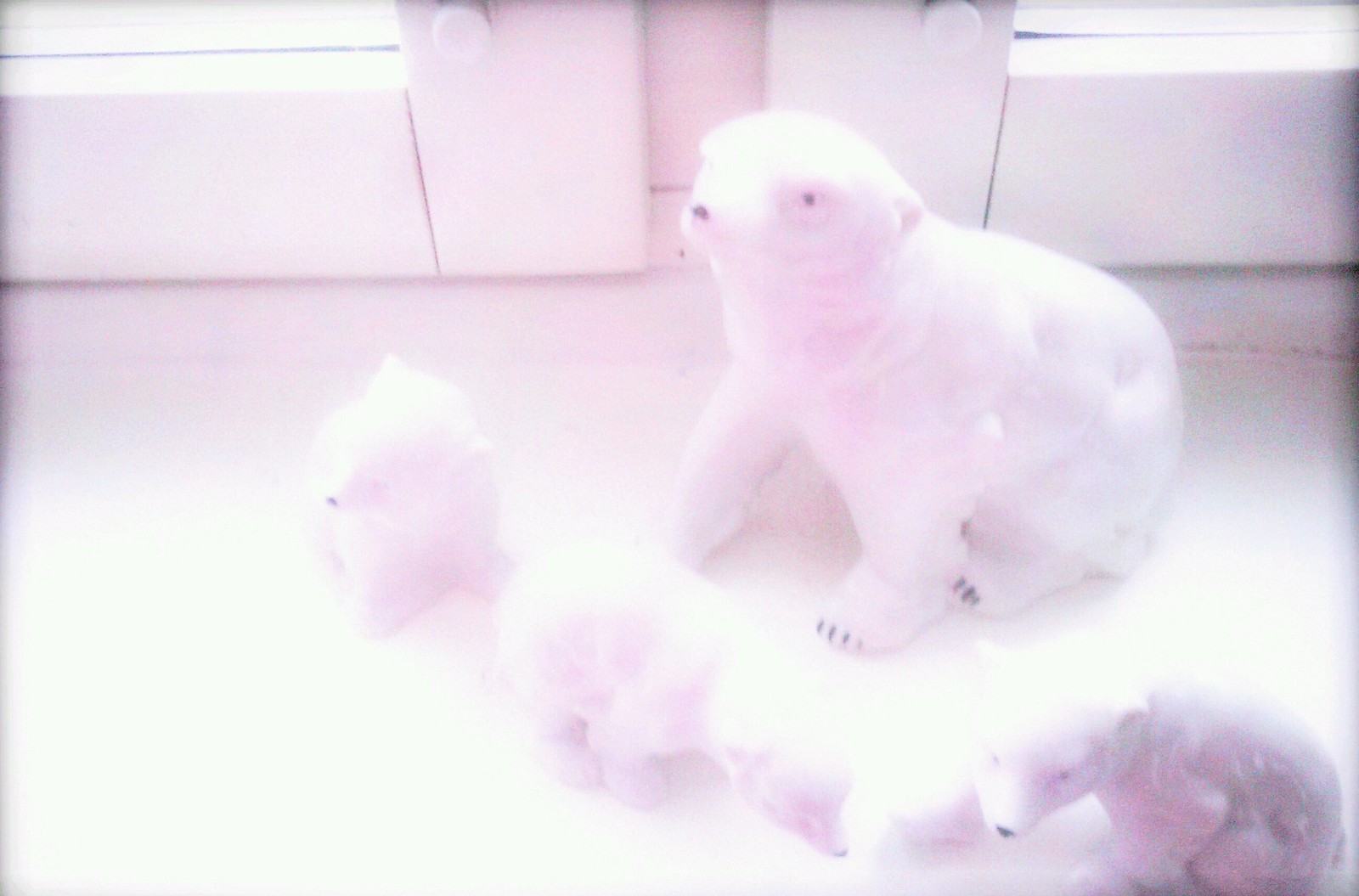This photograph captures an overexposed, overly lit room with an almost ethereal glow, making much of the scene blurred and washed out to the point that white areas blend together. The room features two windows set against white walls, which are flooding the space with intense light, creating a pinkish-purplish tint due to the overexposure. The floor, also white, serves as the stage for a group of white statues, presumably made of stone or marble given their pitted texture. These statues depict a family of polar bears: an adult polar bear with small ears, a black nose, black eyes, and painted black toenails sits with its left leg extended. In front of the adult bear are three baby polar bear statues, each with black noses and small ears. One baby polar bear sits to the left, looking outward, while another sits slightly upright, tucked in on itself. The last baby bear has distinct black eyes and is positioned as if moving its legs forward. The intense exposure erodes the details, giving the statues and the overall scene a somewhat surreal appearance.